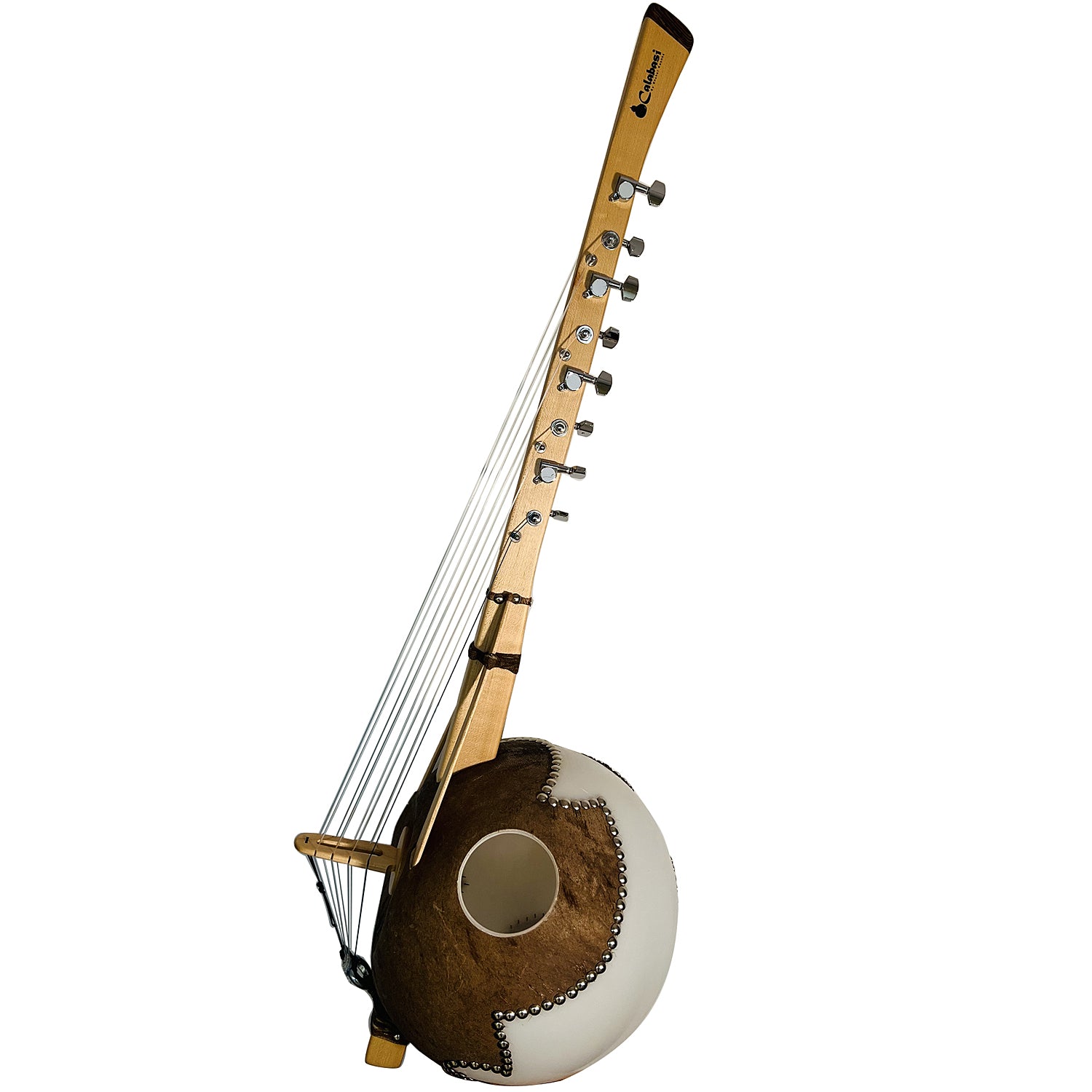This image portrays a unique, possibly vintage musical instrument that may resemble an old type of guitar. The instrument features a long, light brown wooden handle, which darkens towards the top. Notably, the handle appears to have eight tuning clamps or screws aligned along the side, which secure the strings running down its length. The instrument's body is distinctively circular and resembles the size and shape of a coconut; it is primarily dark brown with a white outer shell and has a central hole. The word "Calabassey" is inscribed on the handle, suggesting that this might be the name of the instrument. The image is set against a plain white background with no other objects or text, indicating it might be a retail or catalog photograph.